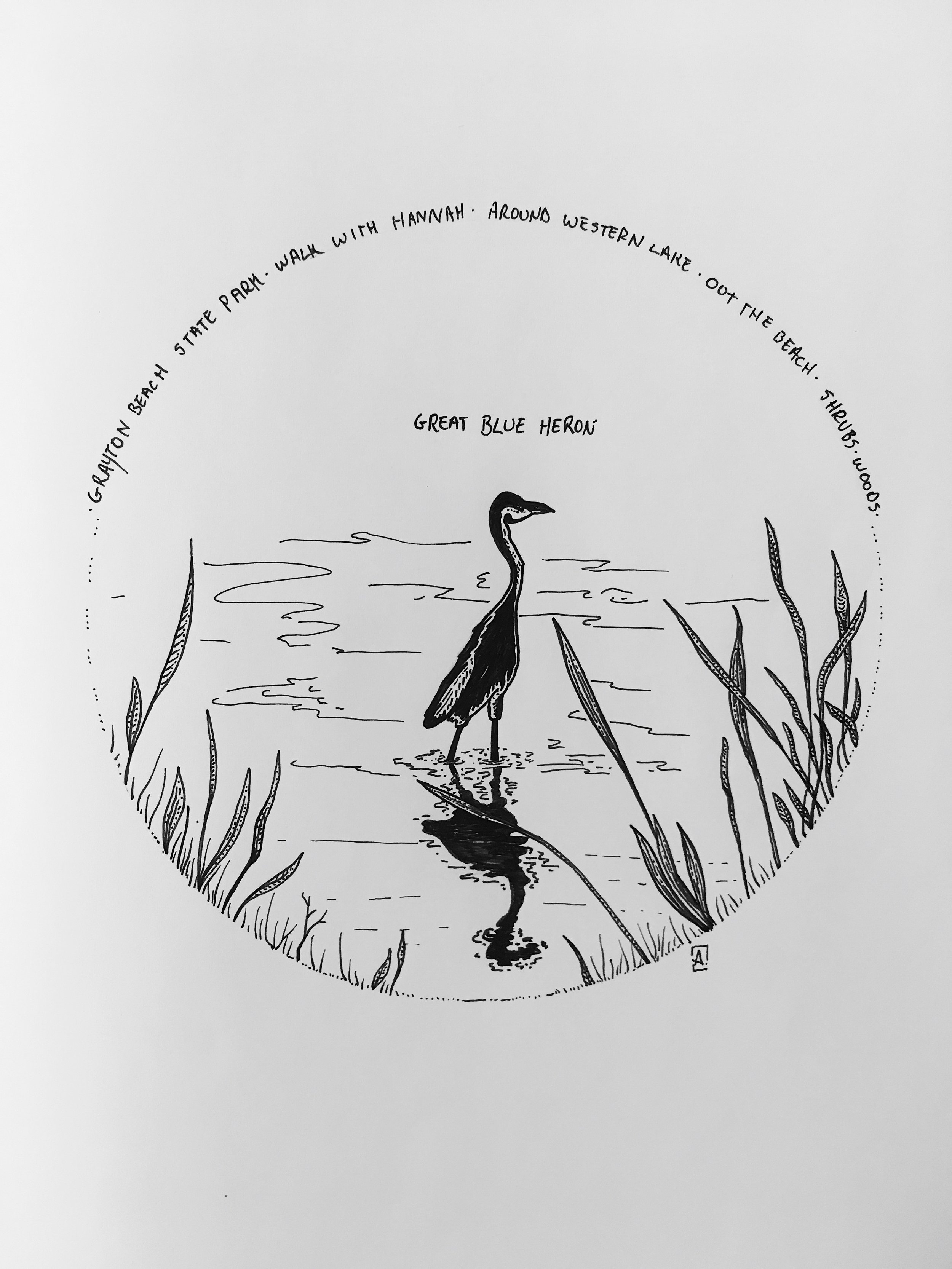In this scientific textbook-style artwork, we see a detailed, hand-drawn illustration of a Great Blue Heron, rendered in black and white, possibly with pencil or charcoal. The image is set within a circular frame and captures the heron standing gracefully in a body of water, with its long neck extended and a short beak pointed to the right. The bird's elongated body and long feathers are meticulously depicted, with its legs partially submerged but notably rising above the water’s surface. Surrounding the heron, various elongated plants and reeds emerge from the water, creating a naturalistic environment.

The circular frame is bordered by text, with an arched caption at the top reading "Grayton Beach State Park. Walk with Hannah. Around Western Lake. Out the Beach, Shrubs, Woods." At the bottom of the circle, the caption states "Great Blue Heron," indicating the species of the bird. Below the heron, its reflection is visibly mirrored in the water. Additionally, there is a small box containing the letter "A," likely the artist's signature, located within the illustration. This carefully crafted image evokes the serene and detailed essence of a scientific illustration with a touch of artistic elegance.